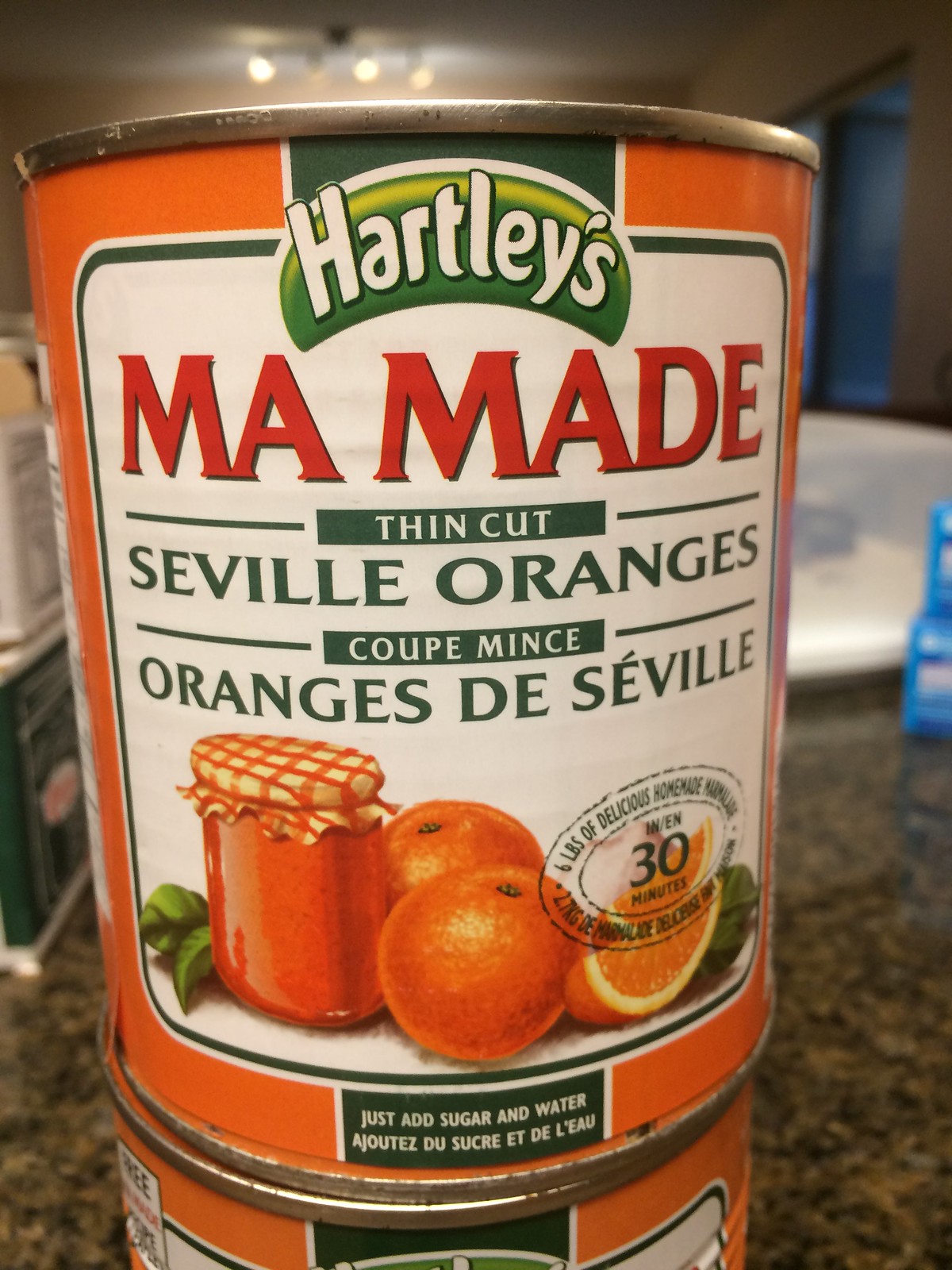This photograph features a vibrant food container resting on a kitchen countertop that combines black and caramel tones. The container is decorated in various shades including green, orange, red, and white. At the top, the brand name "Hartley's" is displayed in white font against a green background. Directly below, the phrase "maw made" appears in red font, followed by "thin cut" in white font, "Seville oranges" in green font, "coupe mince" in white font, and "oranges de Seville" in green font. The container also features an image of orange marmalade with an orange and white covering, surrounded by some fresh oranges. At the bottom, the instructions "just add sugar and water" are written in white font. The background includes other objects that are blurred and indistinct.